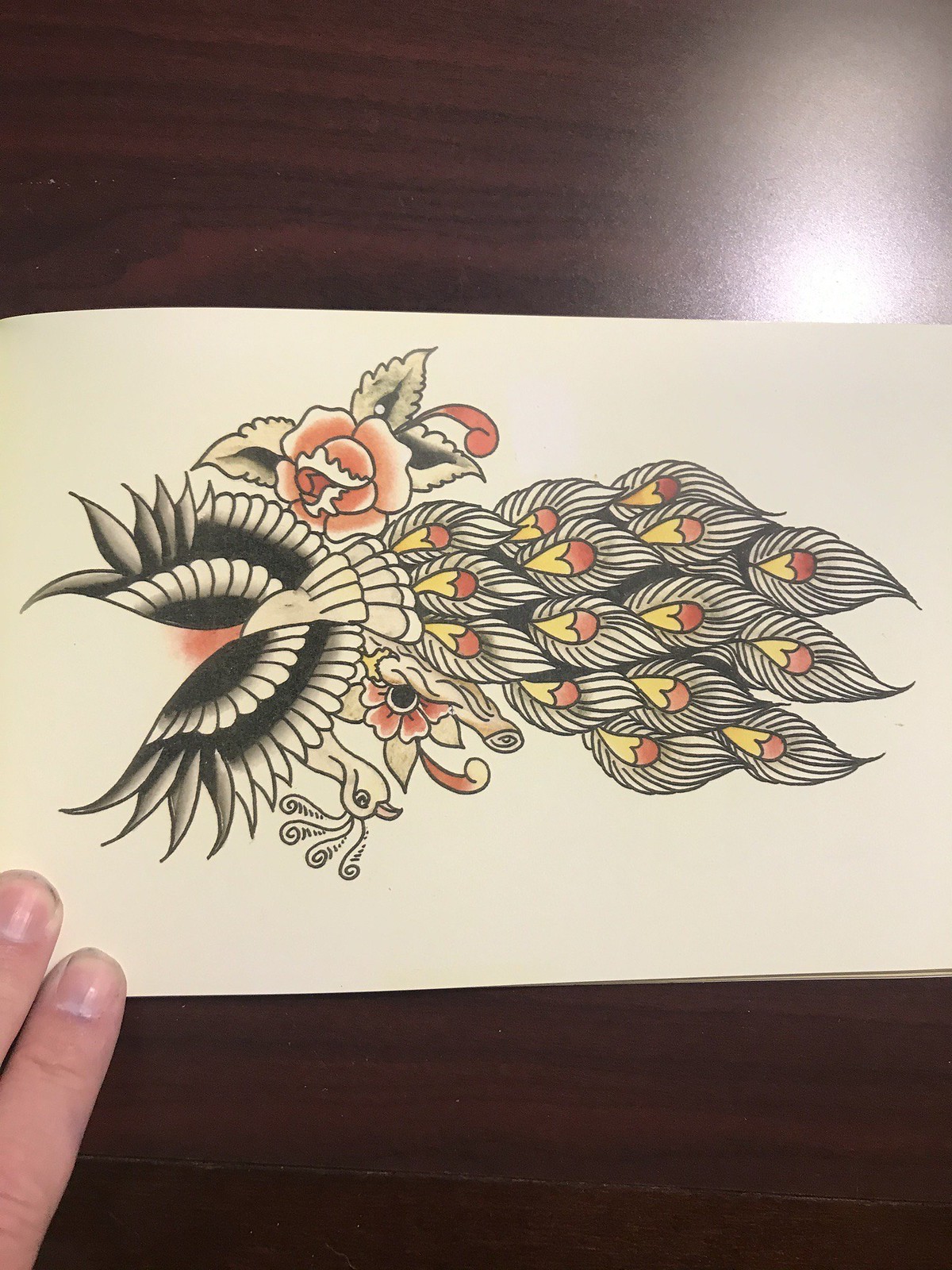A meticulously crafted piece of pen, ink, and marker artwork is resting on a rectangular strip of white paper, which is placed atop a dark walnut tabletop. In the lower left corner of the image, an index and middle finger are partially visible, anchoring the sheet of paper securely. The artwork itself showcases an array of colors, with hues of black, white, cream, orange, yellow, and tangerine brown. These colors are skillfully used to depict peacock feathers that fan out gracefully from the left side of the paper to the right. Each feather is intricately detailed with precise black line work enclosing vibrant centers of yellow and orange. In the bottom left corner, the head of a peacock can be seen, revealing that the paper has been rotated 90 degrees clockwise, causing the bird to appear as if it's lying on its head. The contrast of the vivid artwork against the rich, dark wood of the tabletop enhances the captivating beauty of the piece.